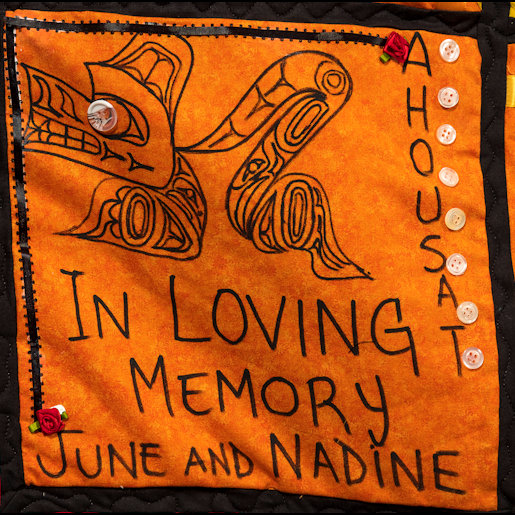The image depicts a slightly wavy, orange square patch, akin to a tile from a quilt, bordered in black. The patch features black lettering at the bottom that reads "In Loving Memory of June and Nadine." Vertically down the right side, the letters "A-H-O-U-S-A-T" are inscribed, accompanied by white and yellow buttons that align with them. The top left corner droops slightly, adding to the undulating texture. Along the top and left sides, a black strip resembling stitches or a zipper spans from the bottom left to the top right, where it overlaps with the inscription. Below this strip are winding line designs reminiscent of stylized snakes with possible teeth. Tiny rose embellishments, like craft roses, appear at the bottom near the names and at each end of the black strip.